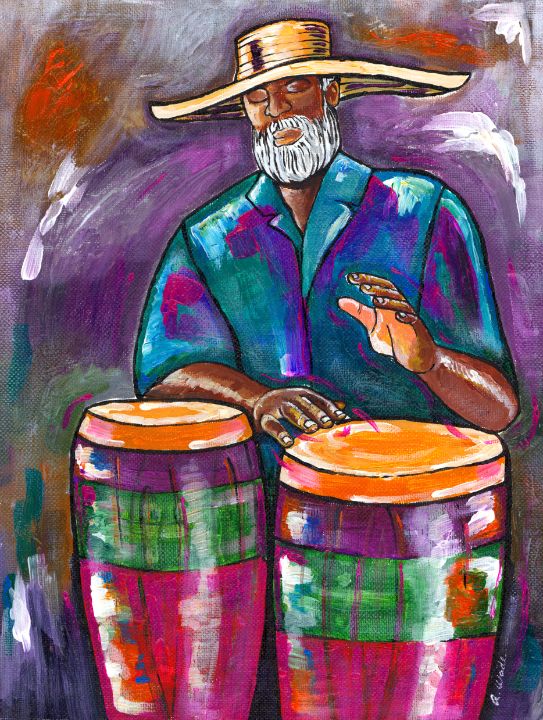The painting titled "The Sound of the Beat" is a vivid and colorful piece in a portrait orientation. The centerpiece is an African-American man with his eyes closed, deeply immersed in playing two bongos. He sports a large woven straw hat and has a distinguished white beard and mustache. His turquoise blue button-up shirt features accents of pink, purple, and blue. The bongos he plays have orange tops, with their bodies adorned in stripes of purple, green, and pink. 

One of the man's hands rests on a bongo while the other is raised, capturing the motion with pink squiggly lines. Surrounding him is a dynamic, swirling background of purples, whites, and oranges, contributing to the energetic yet peaceful vibe of the scene. In the bottom right corner, there is a small, barely legible artist's signature. The man's serene expression and the vibrant colors convey a deep sense of joy and connection to the music.